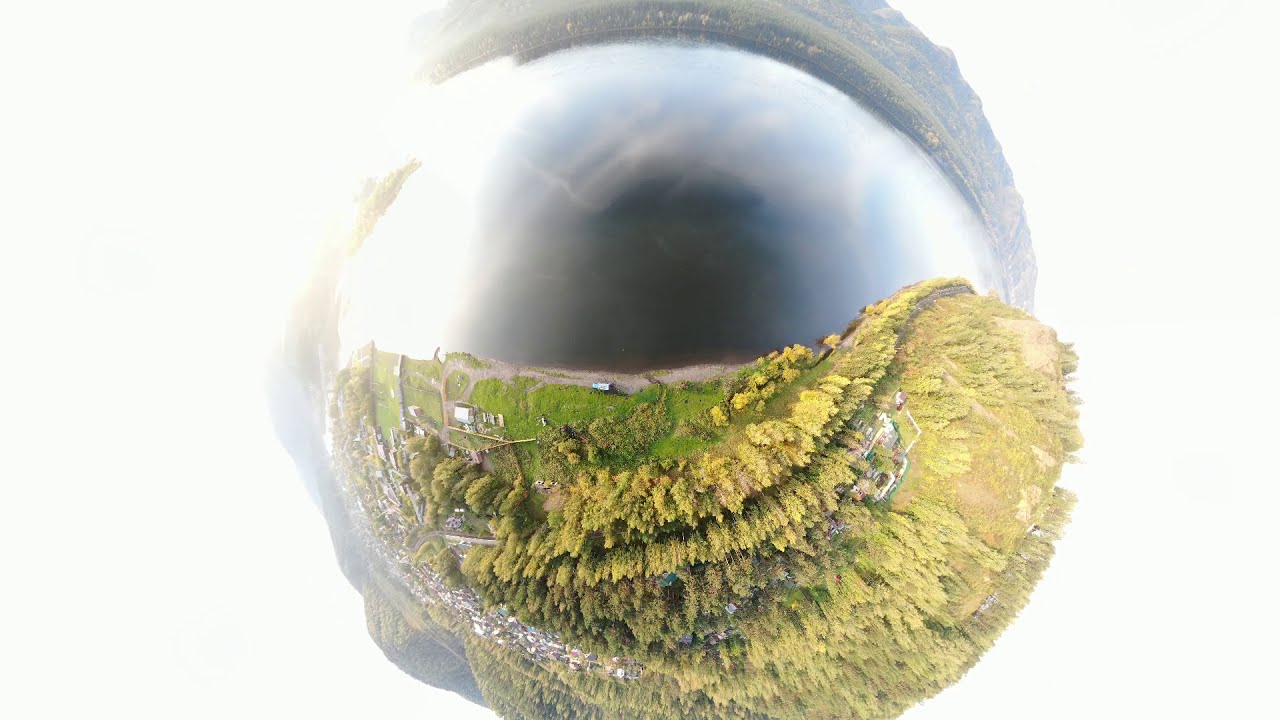This intriguing aerial photograph, captured with a fisheye lens, presents a highly distorted and almost orb-like view of a diverse landscape. Dominating the image are lush, green-yellow trees and vegetation interspersed with patches of green grass. Towards the bottom of the image, the greenery appears to extend outward, resembling an organic growth. The backdrop reveals a mountain range devoid of snow, adding a rugged terrain element to the scene. A small town is faintly visible in the distance, indicating signs of civilization. Closer to the camera, near what appears to be a lake or stream, there's a house and barn positioned next to the water, along with a parked truck roughly 20 feet from the shore. The overall color palette includes shades of green, white, yellow, blue, gray, and black, contributing to the picture's unique and slightly surreal appearance. The background outside the central distorted circle is a bone-white, slightly yellowish tone, enhancing the visual contrast of this fisheye, bird's-eye view composition.